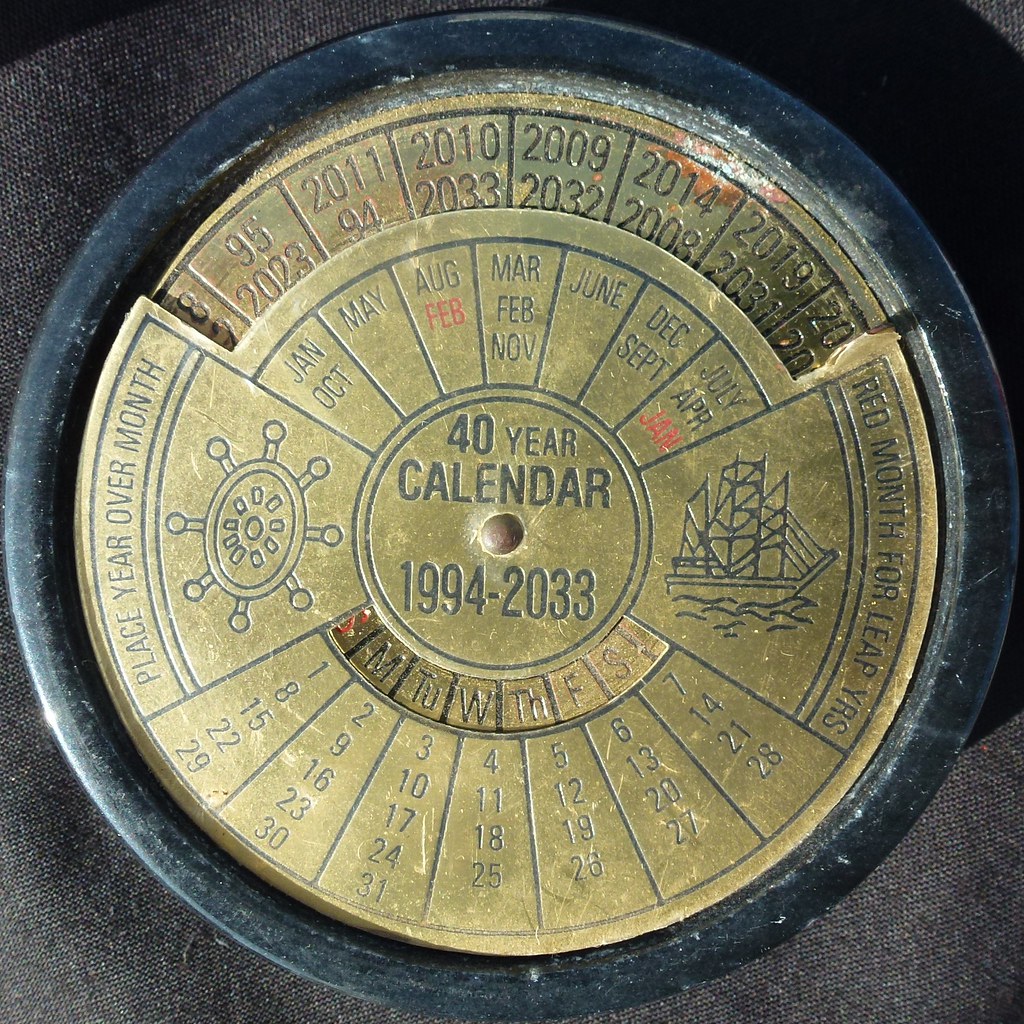This photograph features a detailed metal 40-year circular calendar spanning from 1994 to 2033. The calendar is constructed of two concentric pieces of metal that can be rotated to display various dates. The center disc is gold with black etched writing, encircled by a black frame. Engraved in the very center is "40-year calendar 1994-2033." Surrounding this central text are the months, including January, February (marked twice), March, April, May, June, July, August, September, October, November, and December. Notably, the months of January and February are highlighted in red.

To the left of the center, the inscription reads "place year over month," accompanied by an image resembling a ship's wheel. On the right side, there is a depiction of a ship with the label "month for leap years" in red. Below the central section, the days of the week (Sunday through Saturday) are listed, followed by groupings of days in numerical ranges: 1-7, 8-14, 15-21, 22-28, and 29-31.

At the top edge of the calendar, a series of years are inscribed: 95, 2011, 2010, 2009, 2014, 2019, 2023, 94, 2033, 2032, 2008, and 2031. The photograph also captures a shadow in the top right corner, indicating that the light source is positioned at the bottom left. All engravings on the calendar are in red or black, enhancing its intricate design.